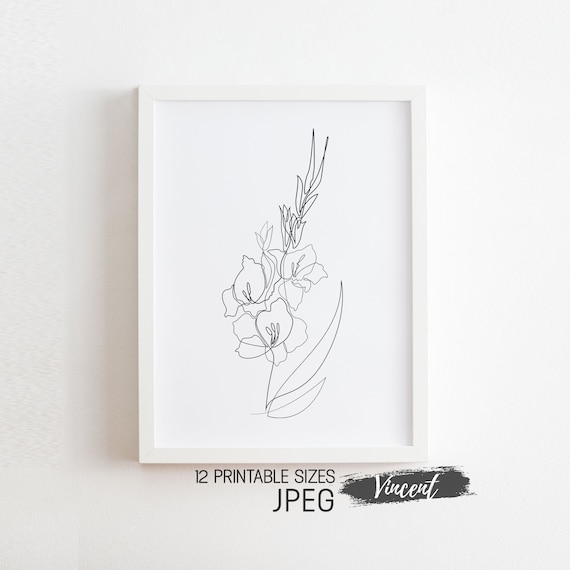This image displays a white, vertically-oriented wooden frame hanging on a white or light gray wall, containing a minimalist ink drawing. The drawing, rendered in a single continuous black line, features a botanical motif comprising a stem emerging from the bottom, topped with two thin leaves—one shorter and one longer—on the right side. Further up the stem, three multi-petaled flowers are depicted: one central bloom with visible inner prongs, flanked by two additional flowers on each side. Above these blooms, additional foliage, including two buds and two thinner leaves directed upwards and to the right, completes the composition.

Below the drawing, there is text in a regular font that reads "12 printable sizes, JPEG." In the bottom right-hand corner under the frame, a dark gray brush stroke serves as a backdrop for the artist's signature, "Vincent," rendered in white cursive letters. This delicate sketch emphasizes simplicity and elegance, capturing the essence of flowers with minimal detail and no shading.